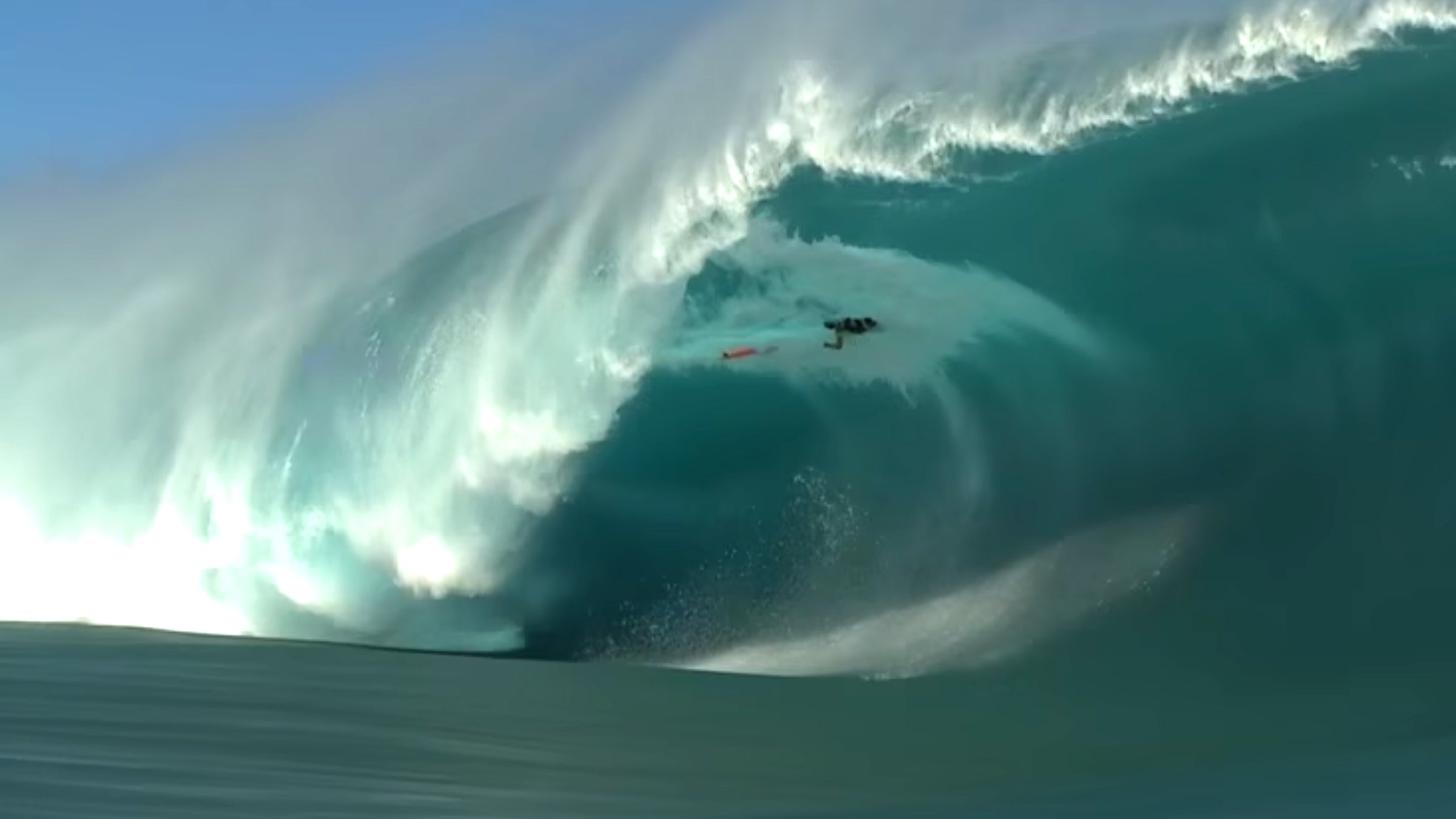This photograph captures the dramatic scene of an enormous wave in the ocean, caught mid-crest with its formidable circular motion dominating the frame. The wave, towering about 10 people high, presents a powerful display as it transitions from smooth, flat water on the far left to a majestic curve that swoops up and over. The surface of the wave is a striking greenish hue, with white froth where the water crashes and churns. The top edge of the wave is fringed with a white rim, indicative of the immense energy it carries. 

Halfway through the picture, toward the top, we see two surfers, one dressed in black and another marked by an orange detail, possibly the surfboard. They appear minuscule against the grandeur of the wave, emphasizing its sheer size and scale. The photograph is taken from afar, providing an expansive view that captures both the cresting peak and the smooth expanse of the ocean below. The sky peeks through only in the upper left corner, adding a touch of blue to the overwhelming presence of the colossal wave.